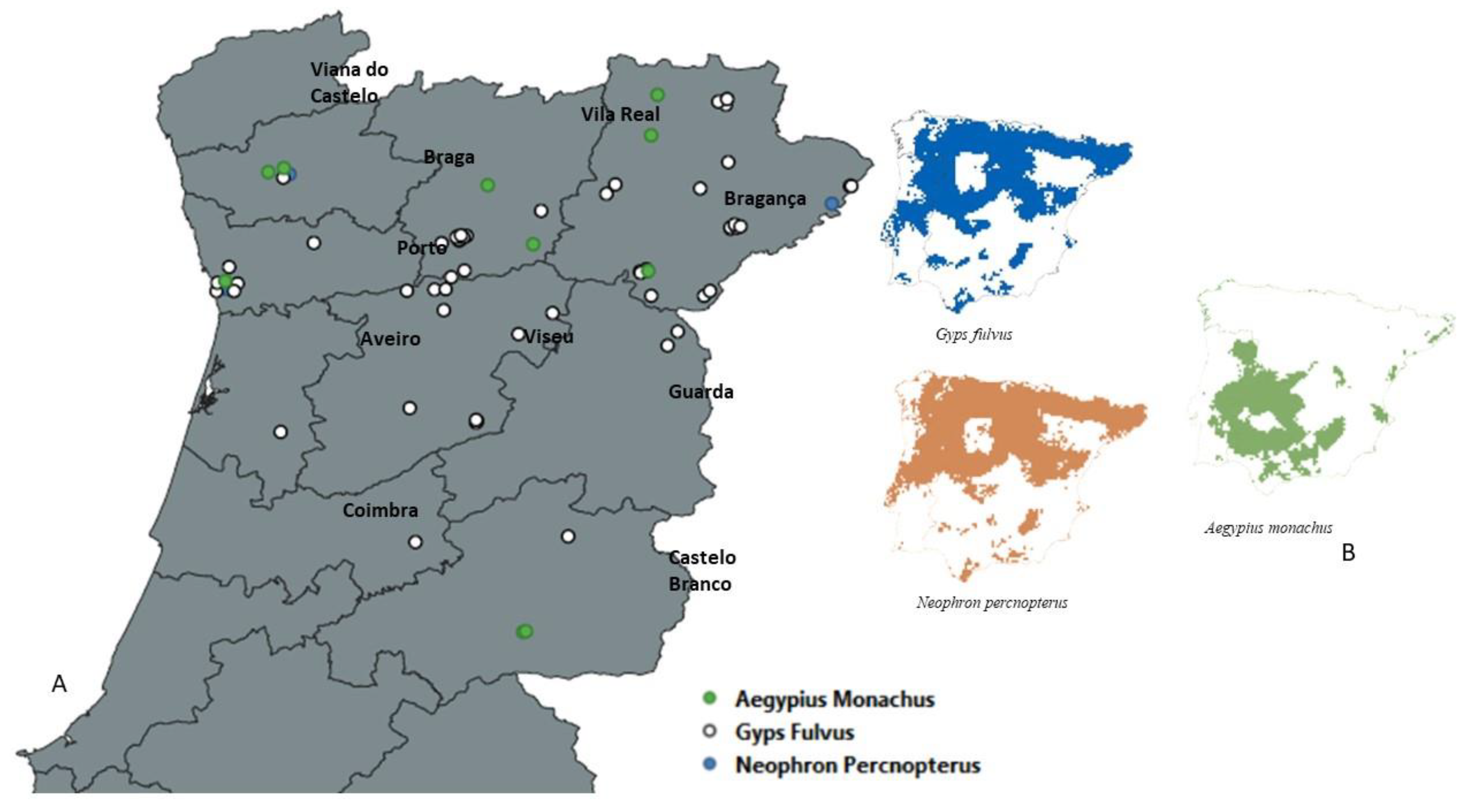The image features a detailed map focused on a European region, likely Portugal, given the city names such as Coimbra, Aveiro, Braga, Porto, Viana do Castelo, Guarda, and Castelo Branco labeled in black font. The main map, predominantly gray, is sectioned into titled regions, with green and white dots marking specific locations within these areas. Surrounding the main map are three auxiliary illustrations: to the left is a dense blue-colored map, below it an orange-brown map with varying densities, and to the right a green map with both dense areas and scattered green spots. These additional maps likely represent different data distributions or thematic layers related to species or ecological zones in the region.